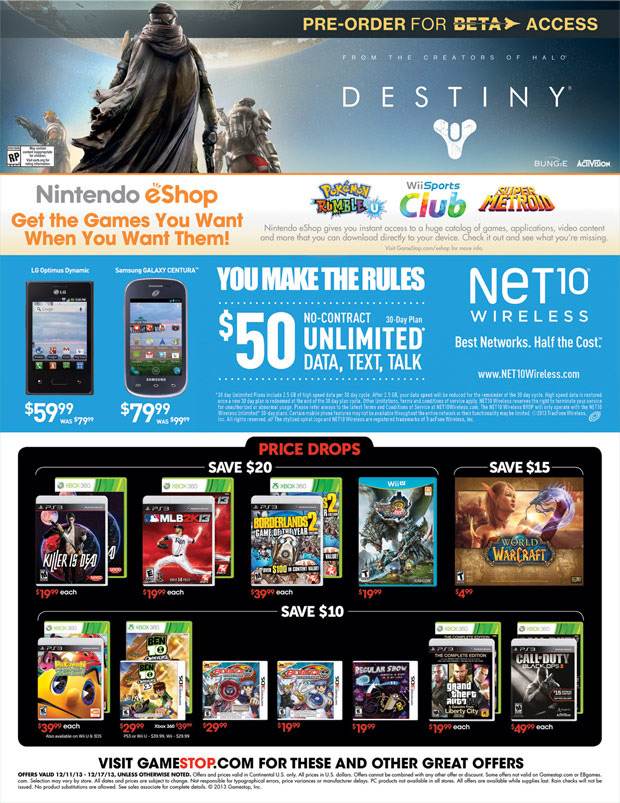Set against a pristine white background, the image appears to be a promotional poster reminiscent of something from a movie or a video game. At the top right, vibrant yellow text urges viewers to "pre-order for beta access," with an adjacent white text endorsement highlighting, "From the creators of Halo, Destiny." Further down, the lower right prominently displays "Activision" in white text, reinforcing the credibility of the advertisement. Centered below this, an orange and gray banner proudly proclaims, "Nintendo eShop" on the left in gray, followed by the inviting message in orange, "Get the games you want when you want them."

Beneath, a blue banner showcases a selection of electronic advertisements. On the left, an image of a compact tablet is marked with the label "LG Optimus Dynamic, $59.99" in clean white text. Adjacent to it, a sleek cell phone, identified as the "Samsung Galaxy Centura," is priced at $79.99. To the right, bold white text assures customers, "You make the rules," highlighting an attractive offer of "$50 unlimited data, text, talk."